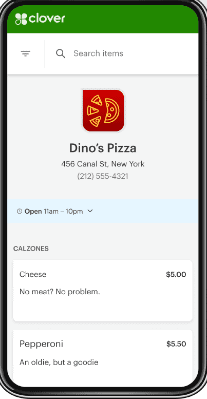This screenshot, captured from a smartphone, showcases a section of the Clover app, identified by its green banner featuring a white logo with the inscription "clover" and a four-leaf clover. Notably, three of the clover's leaves are colored white, while the bottom left leaf remains uncolored.

This particular section highlights a restaurant named Dino's Pizza, recognized by its red square logo incorporating an orange pizza outline. The pizza design is partially solid, with the other half segmented into three slices. Below the logo and the restaurant name, the address "456 Canal Street, New York" is displayed, accompanied by a contact phone number.

The screenshot provides a glimpse of the restaurant's operating hours and a portion of its menu, spotlighting two items: a Cheese Calzone and a Pepperoni Calzone. Each item has a brief, engaging description and corresponding price. The Cheese Calzone, priced at $5, is described with the tagline "No meat, no problem," while the Pepperoni Calzone, priced at $5.50, is labeled affectionately as "An oldie but goodie."